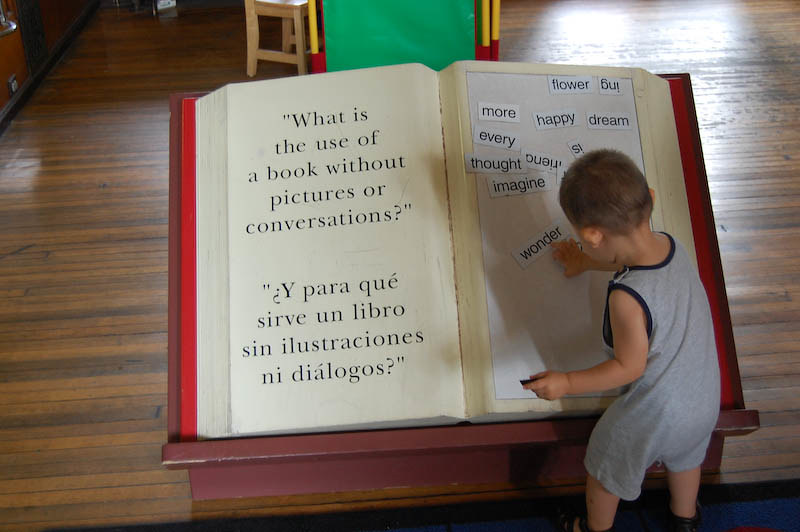In this horizontally aligned, color photograph, a very young toddler boy, possibly between one and a half to two and a half years old, stands at the bottom right corner. The boy is dressed in a gray onesie with blue trim and black sandals, and has brown hair. The scene depicts him interacting with an oversized playbook set on a podium that stands taller than him. The book is open, revealing a two-page spread. On the left page, in black text over white paper, it reads: "What is the use of a book without pictures or conversations?" followed by the Spanish translation: "Y para qué sirve un libro sin ilustraciones y diálogos." Both sentences are in quotation marks.

The right page of the book is designed for pasting words, and the young boy is engrossed in sticking the word "wonder," a white label with black text, onto the page. Other visible words already pasted onto the page include "flower," "buy," "more," "happy," "dream," "every thought," "imagine," and "wonder." The child is captured from behind, with his right hand touching the word "wonder" and his head turned downwards, focusing on his task. The background reveals a wood plank floor in shades of dark and medium brown, with partial views of tables near the top of the image. The photograph is a perfect representation of a serene and imaginative moment, blending in elements of play and learning.